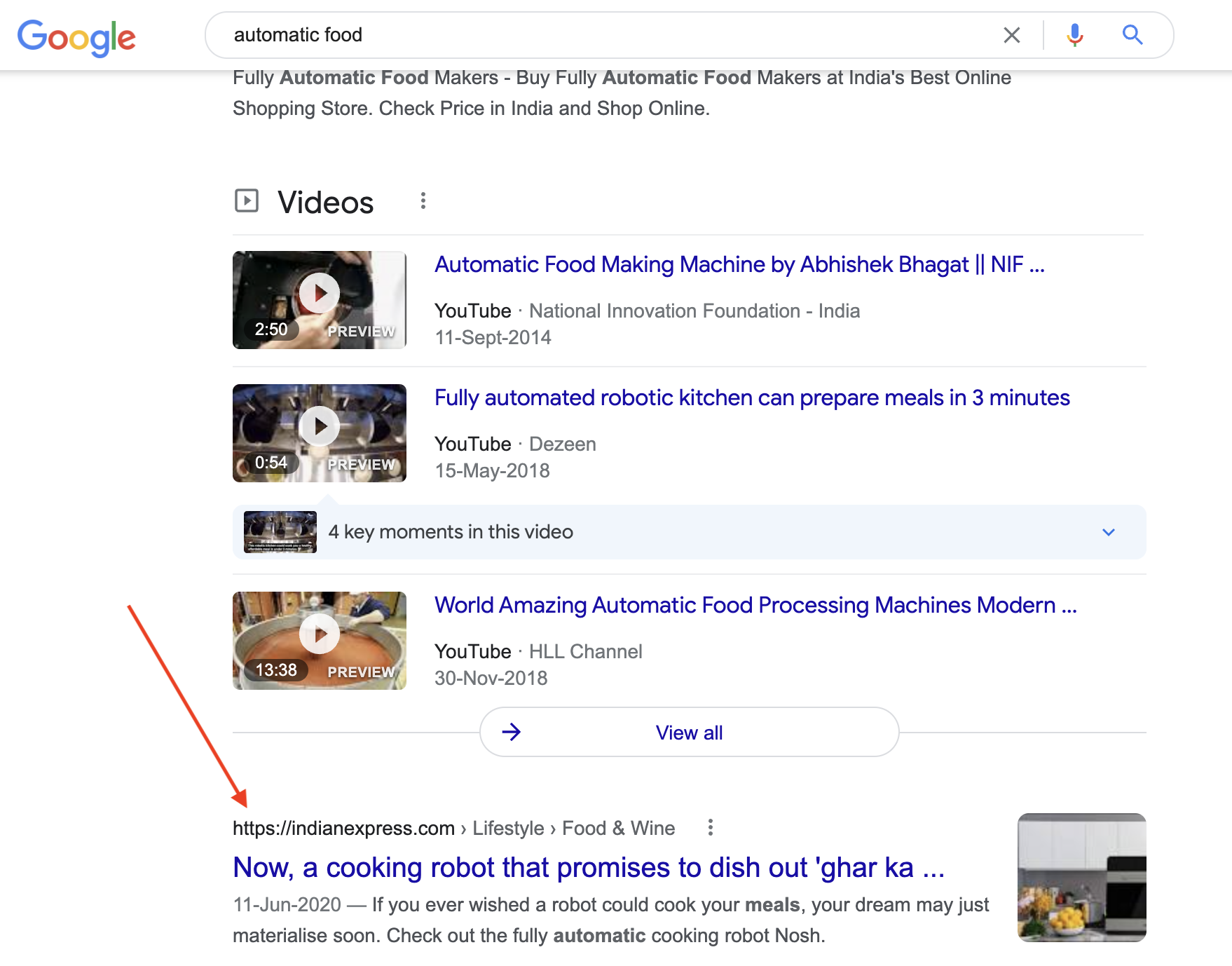Here is the cleaned-up and detailed caption:

---

This image captures a Google search results page. The familiar Google logo, featuring the colors blue, red, yellow, and green, is displayed in the upper-left corner. In the search bar, the user has entered the query “automatic food.” Adjacent to the search bar, there is a microphone icon in Google colors, an 'X' button, and a magnifying glass icon representing the search function.

Below the search bar, the first search result headline reads: “Fully automatic food makers. Buy fully automatic food makers at India's best online shopping store. Check price at India and shop online.” Underneath the headline, tab options like "Videos" are visible, indicating content categorization.

The first video result is titled "Automatic Food Making Machine," uploaded by the YouTube channel “National Invention Foundation India” on September 11, 2014. It features a white circle with a black play button icon in its center. 

The second video result is titled “Fully Automated Robotic Kitchen Can Prepare Meals in Three Minutes,” uploaded on May 15, 2018, also showing the play button icon. 

There is a light blue bar labeled “Four key moments in this video,” highlighting important video segments. Below this, a section titled “World Amazing Automatic Food Processing Machines Modern” features an image of a large pot of soup with a white play button icon overlaid. It provides an option to “Preview all.”

At the bottom, a red arrow points towards a website, accompanied by text promoting a cooking robot promising to deliver homemade-style dishes: “Now a cooking robot that promises to dish out gar ka.”

---

This description provides a detailed overview of the elements within the image and organizes the information more clearly.